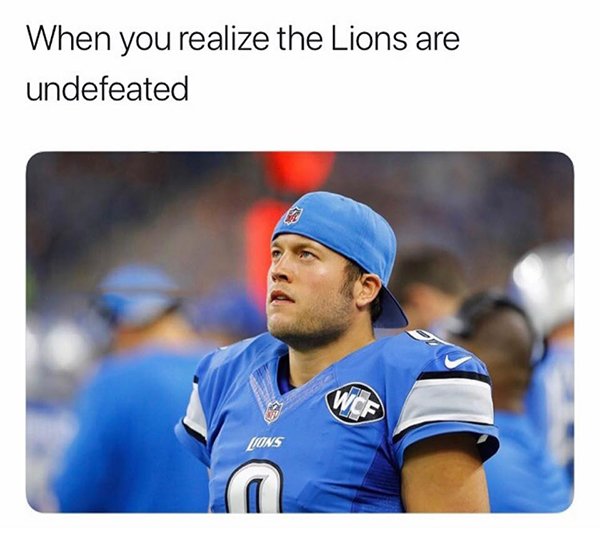The image is a photograph with a white banner on top that has black text reading, "When you realize the Lions are undefeated." Below the banner is a photograph of a Detroit Lions football player, visible from the lower chest upward. The player is clad in a light blue football jersey with discernable bulges from the pads beneath. Near the collar of the jersey, the word "Lions" is printed in white text. The player dons the number nine, presented in white with a black border, on both the shoulder pad and chest. The jersey sleeves feature silver stripes. The player, potentially quarterback Jared Goff, is wearing a baseball cap with the bill pointed backwards, and the back of the cap displays the letters "NFL," indicating it belongs to the National Football League. His face and body are oriented towards the top left corner of the image. The letters "WCF" can be seen on his shoulder, adding to the detailing of the jersey.